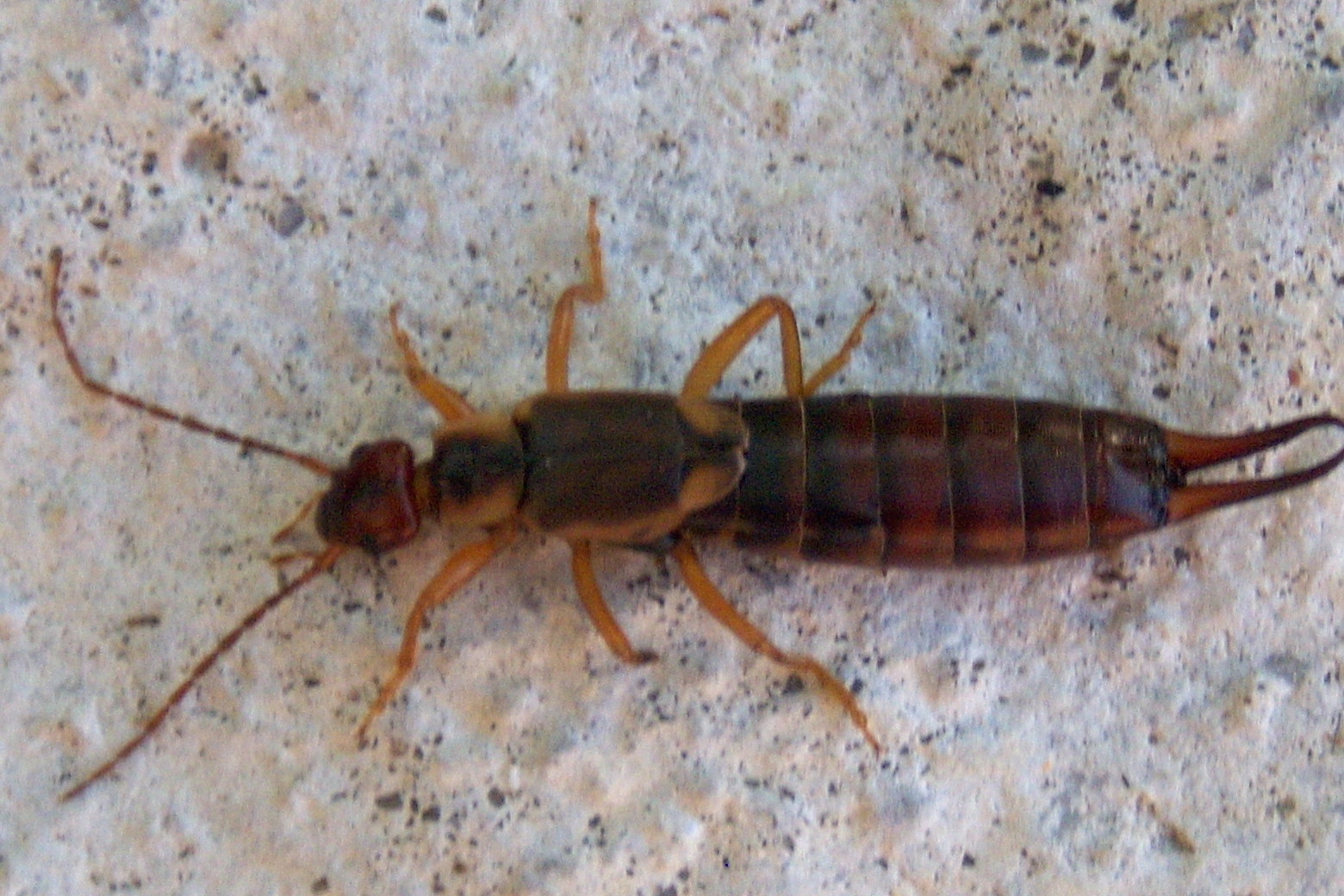This is a close-up photo of an insect situated on an uneven, porous, white rocky surface with specks of gray, peach, and possibly pinks. The insect appears to be alive due to its "meaty" appearance and is predominantly brown-orange in color. It has a reddish-brown head with two long, red antennae extending from it, and six thick, yellowish legs—three on each side. The insect's midsection features dark brown and black hues, transitioning into a segmented abdomen with six distinctive segments. The final segment ends in two pointy orange prongs, reminiscent of a scorpion's pincers. The insect's body has a translucent beige quality in places and its overall length is approximately two inches, making for a strikingly detailed and almost unsettling image on the irregular, countertop-like surface, possibly granite.